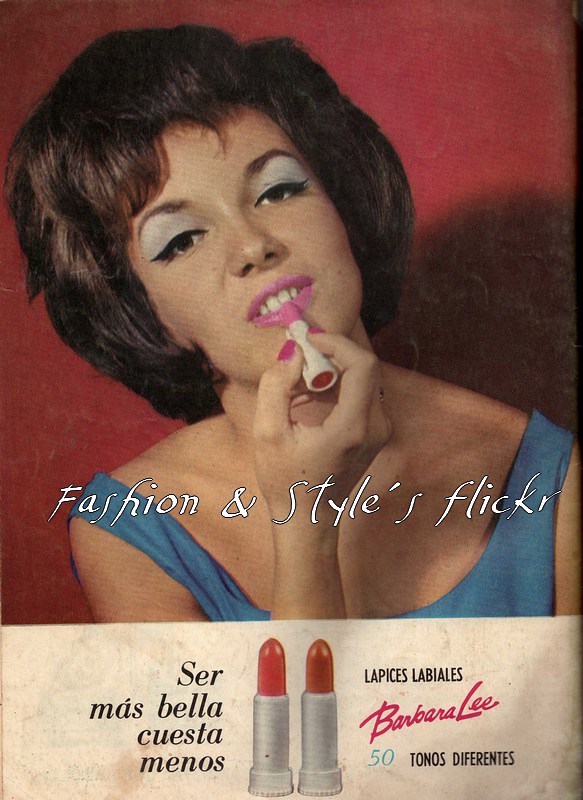The image is a scan of a vintage magazine ad featuring a woman with a 60s or 70s style look. Against a striking red background, she is seen from the chest up, wearing a blue sleeveless dress. Her short brown hair is styled in a bushy manner that frames her face, which is accented with bluish eye shadow on her upper eyelids and hot pink lipstick that she is in the process of applying. The photograph gives a nostalgic feel, emphasizing the era's distinctive fashion.

At her collarbone, white text reads "fashion and styles flicker." Below the photograph, a thick white section showcases two lipstick applicators set against the continued red background. The lipsticks, one a lighter red and the other a darker shade, emerge from silver canisters. Sleek black text on this section states "Sara Masabella, Suesta Menos," followed by "Barbara Lee" in pink. Additional black text reads "50 tonos diferentes," suggesting the availability of 50 different tones.